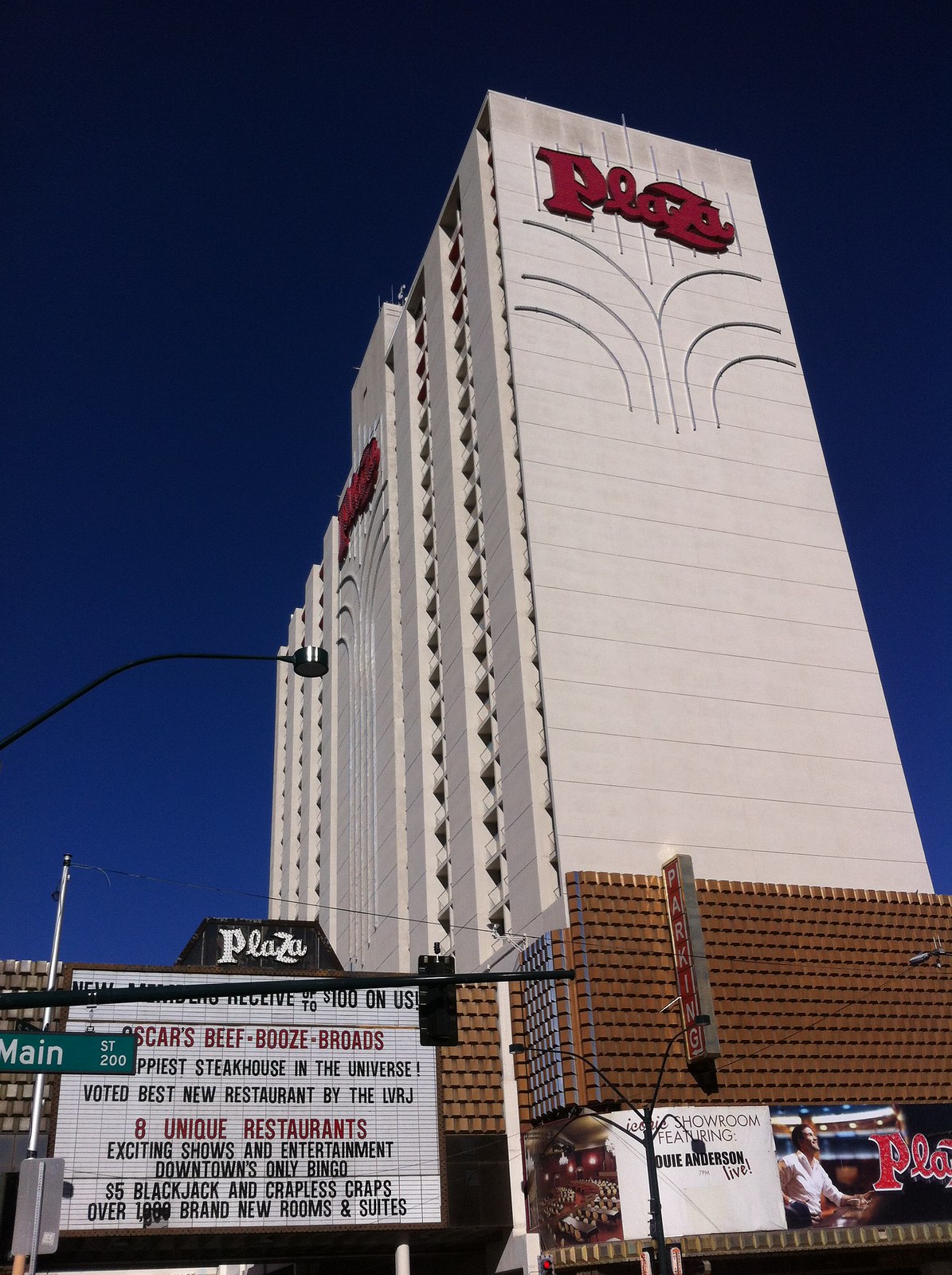This photograph captures a tall, cream-colored hotel building adorned with many balconies, taken from a vantage point across the street. The sky behind the hotel is a deep blue, enhancing the grandeur of the structure which spans several stories. Prominently displayed in cursive red letters on the side of the building is the word "Plaza." Below the hotel, there's a series of brown wooden structures featuring a marquee that advertises various attractions: "Oscars, Beef, Booze, Broads," "Happiest Steakhouse in the Universe," and "Voted Best New Restaurant by the LVRJ." This marquee also highlights amenities such as eight unique restaurants, exciting shows and entertainment, downtown's only bingo, $5 blackjack and crapless craps, and over a thousand brand new rooms and suites. A green pole labeled "Main Street" indicates the location, adding to the vibrant, outdoor cityscape of the scene.